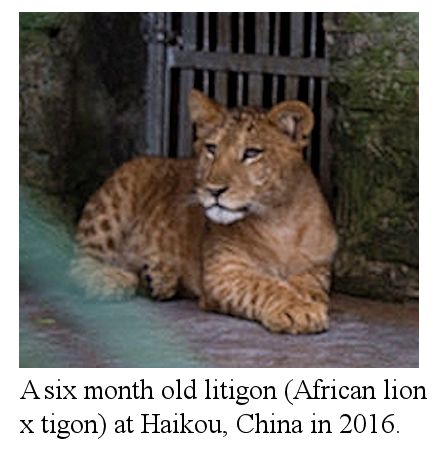This grainy, close-up image features a six-month-old litigon, a cross between an African lion and a tigon. Snapped in 2016 at a holding facility, likely a zoo, in Haikou, China, the litigon is depicted sitting down at the back gate of its cage. Though the picture is slightly out of focus, its unique markings—cheetah-like spots combined with faint tiger stripes—are visible. The young litigon, appearing somewhat disinterested and sleepy, gazes off to the right with its right paw resting forward, positioned in a dirt-floored enclosure adorned with mossy stones. Despite the graininess, the animal's exotic beauty and regal demeanor are unmistakable.